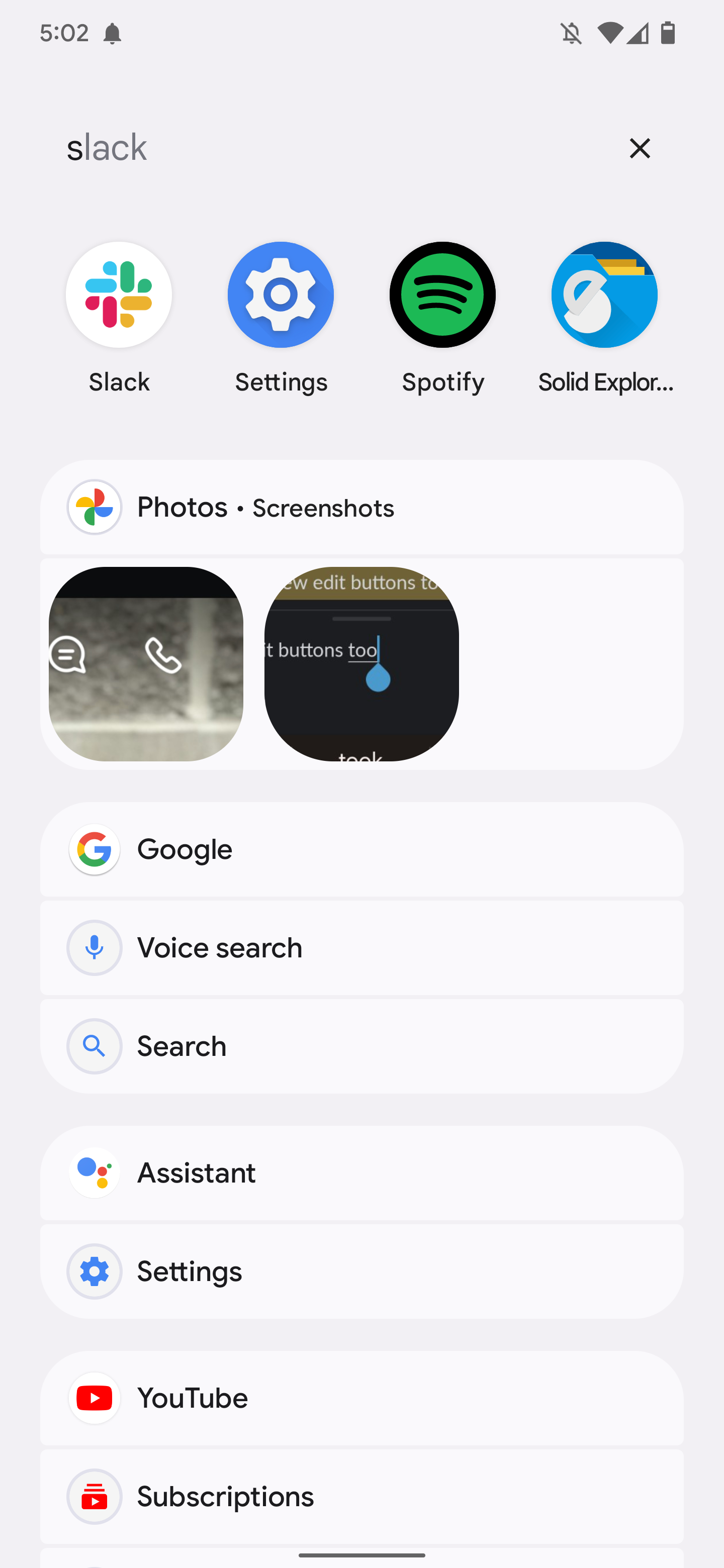The screenshot appears to be from a smartphone, as indicated by several key interface elements present in the image. In the upper left-hand corner, the time is displayed as 5:02, accompanied by a small bell symbol next to it, suggesting there may be an alarm set. To the right, there’s a bell with a line through it, likely indicating that the phone is in silent or do-not-disturb mode. Adjacent to these icons, there is a strong signal indicator followed by a battery symbol showing approximately 75% charge.

Below these status indicators, the interface prominently features the Slack app, a popular collaboration tool similar to Zoom, with its icon displayed centrally. Alongside Slack, there are icons for other apps: Settings, Spotify, and Solid Explorer, the latter of which is a less common file management application. Further down, the Google Photos icon is visible, with a label indicating that there are two saved screenshots.

At the bottom section, there is a series of tabs including Google, Voice Search, regular text search, Assist, Settings, YouTube, and Subscriptions, offering various functionalities and quick access points for the user. The layout and arrangement of these elements suggest a well-organized and actively utilized device, designed for productivity and media consumption.